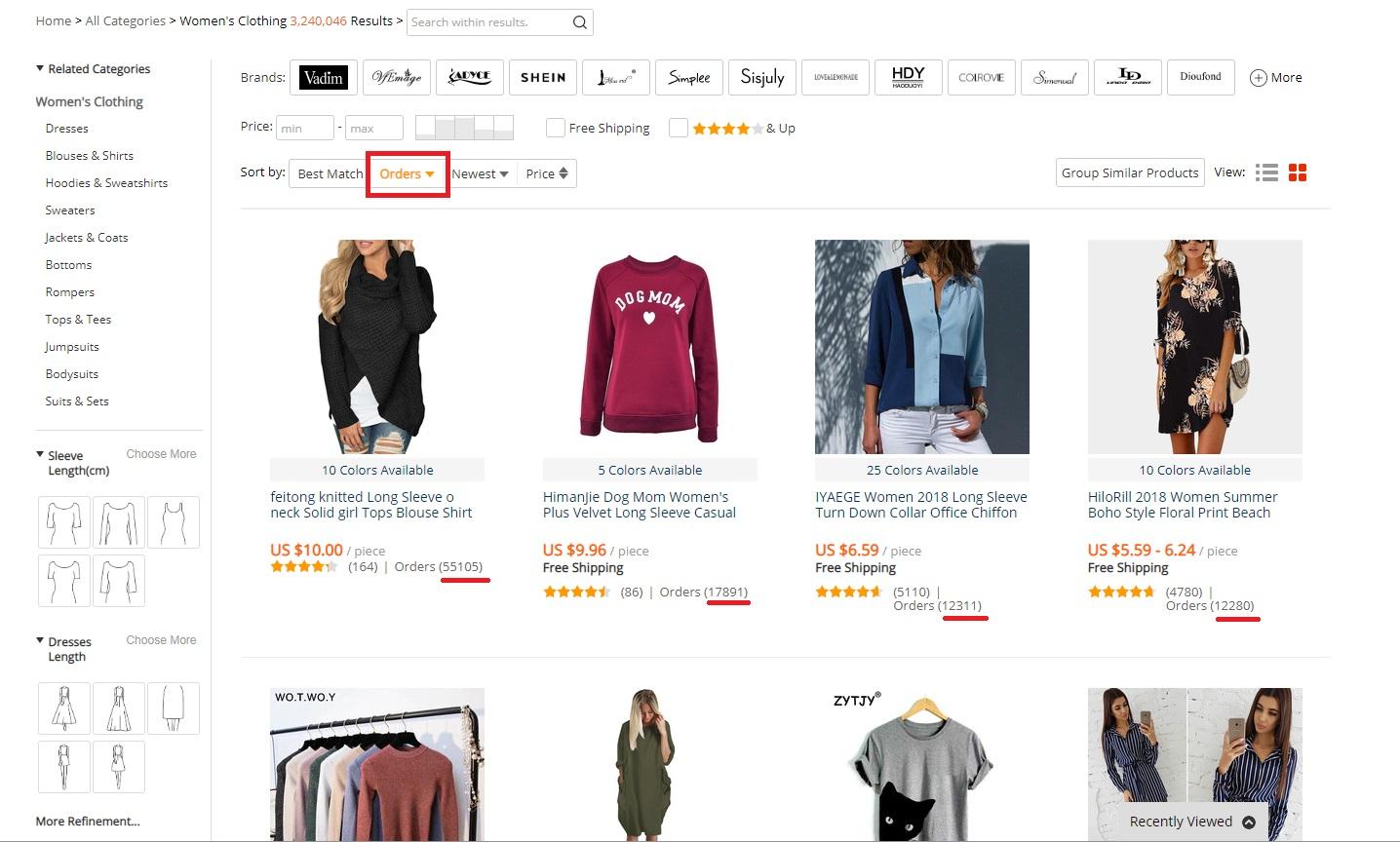"This screenshot depicts an online clothing store page that, at first glance, does not clearly reveal its identity. The top of the page features a horizontal navigation bar filled with numerous brand names, such as Vadum Vintage, Machine, Simply, Sis Julie, HDY, among others. On the left side, a vertical sidebar showcases various categories tagged for easy navigation. These include women's clothing, dresses, blouses and shirts, hoodies and sweatshirts, jackets, coats, bottoms, rompers, tops and tees, jumpsuits, bodysuits, and suits and sets. Additionally, there are options available for selecting sleeve length and dress length. To the right of these category tags is a displayed list of various items, seemingly part of the orders section, indicating that these are products that have been ordered by customers."